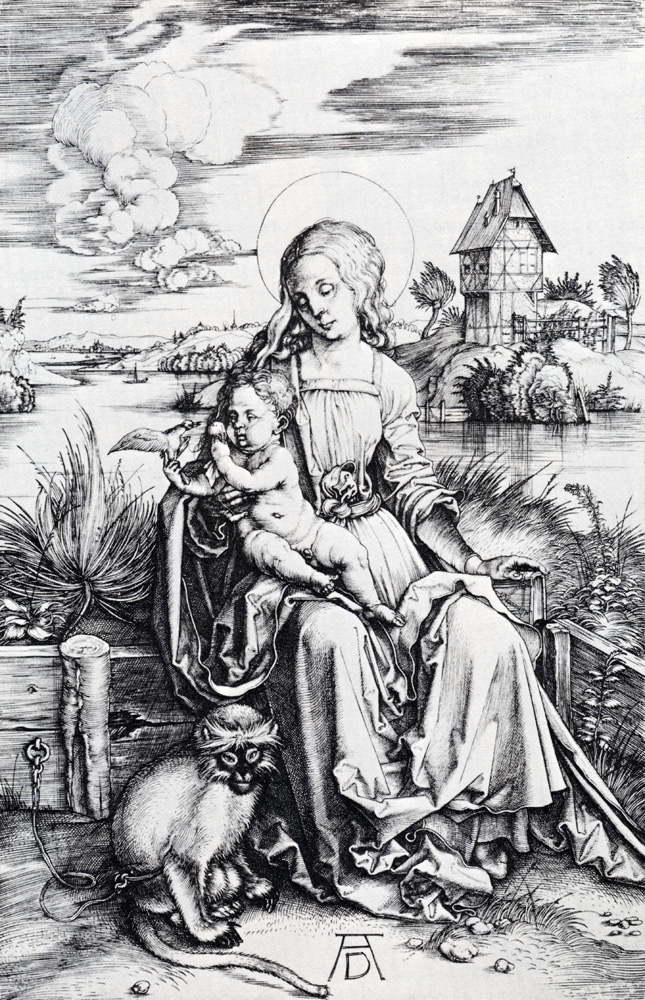This is a highly detailed black and white ink drawing of a seated woman holding a naked, chubby male child on her lap. The woman, who might be depicted as a saint due to the halo encircling her head, wears a long, old-fashioned dress with a square collar that flows past her ankles, obscuring her feet. She has long, wavy, light-colored hair and gazes down at the child, who is leaning to the right, holding a bird in his right hand and interacting with it using his left. At their feet sits a monkey with a long tail and very furry eyebrows, possibly chained to the low wooden wall on which the woman is sitting. Behind them stretches a grassy area leading to a body of water, with an overcast sky filled with clouds above. Far across the water lies a quaint European-style, two or three-story house surrounded by trees and a wooden fence. In the distance, there is a sailboat or fishing boat visible on the water. The drawing is signed at the bottom with the initials "A.D."